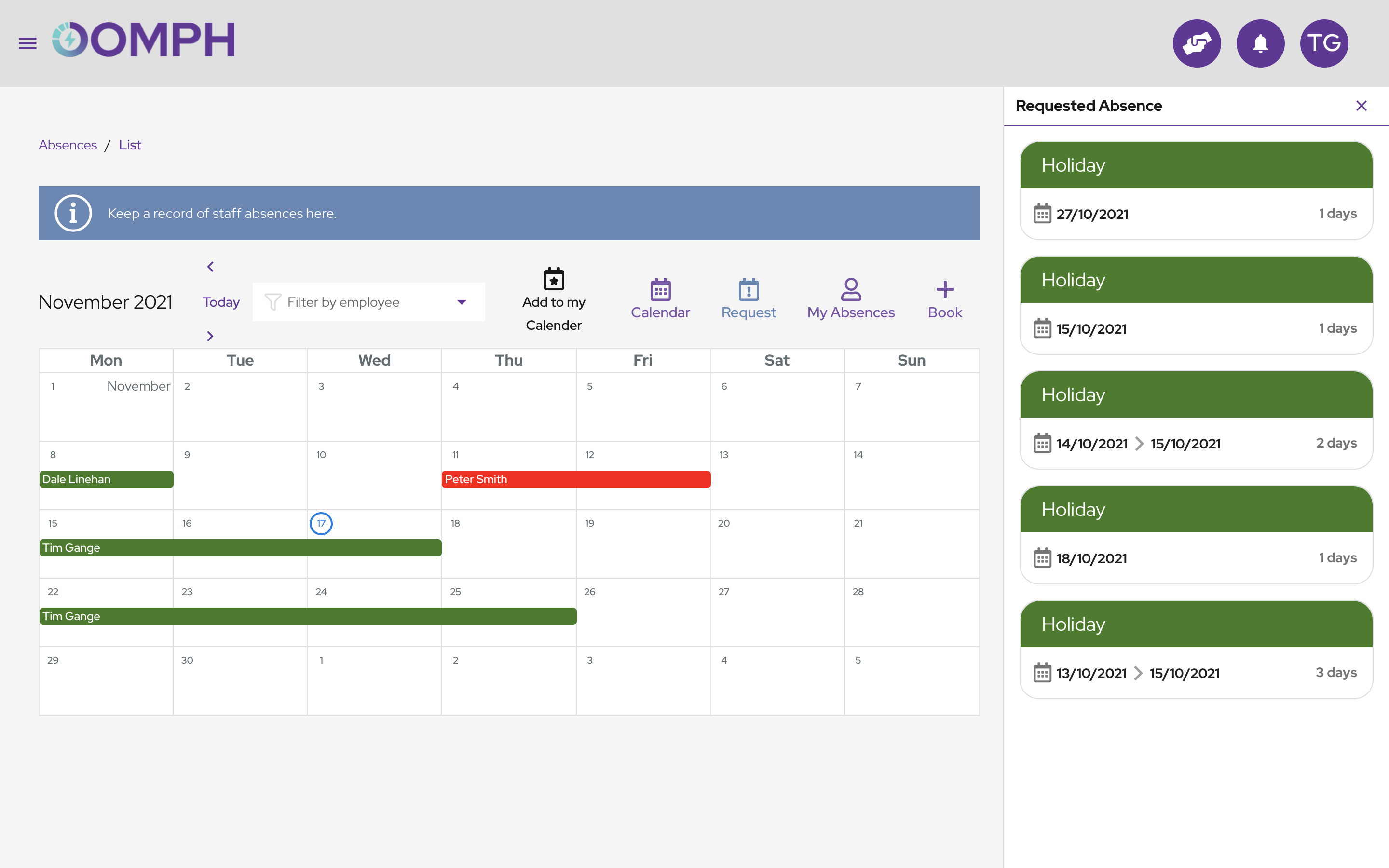In this detailed image of a digital calendar, various elements are meticulously displayed. At the top left corner, there is a notable emphasis on the word "oomph." Below it, links such as "absences" and "lists" are clearly visible. The text prominently highlights the purpose of this interface: "Keep a record of staff absences here." Dates are clearly marked, with the current date highlighted as November 17th, 2021.

Additional options like "filter by employee," "add to my calendar," and "request" are accessible, indicating functionalities for managing and organizing absences. Noteworthy sections such as "my absences" and "calendar book" are also part of this interface. The calendar showcases different entries highlighted in red and green, providing a visual indication of different statuses.

Names of employees such as Peter Smith, Dale Linhan, and Tim Gange are listed, associated with specific events. Notable events include recorded holidays and requested absences, giving a clear overview of the staff schedule for the specified period.